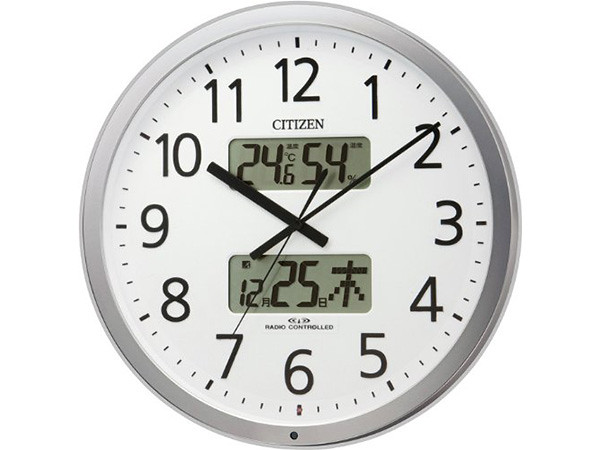A detailed caption for the described image could be:

"A round clock with a sleek silver border features a white face displaying black numbers from 1 to 12, with small black notches marking the minutes. The brand name 'Citizen' is prominently printed on the clock face. In addition to the standard clock hands, which are also black, a digital display shows the ambient temperature as 24.6°C and the humidity level at 54%. The clock includes Japanese kanji characters next to what appears to be calendar dates. Below the kanji, the words 'Radio-Controlled' are printed in black text, indicating that the clock might be synchronized with a radio signal for accurate timekeeping."